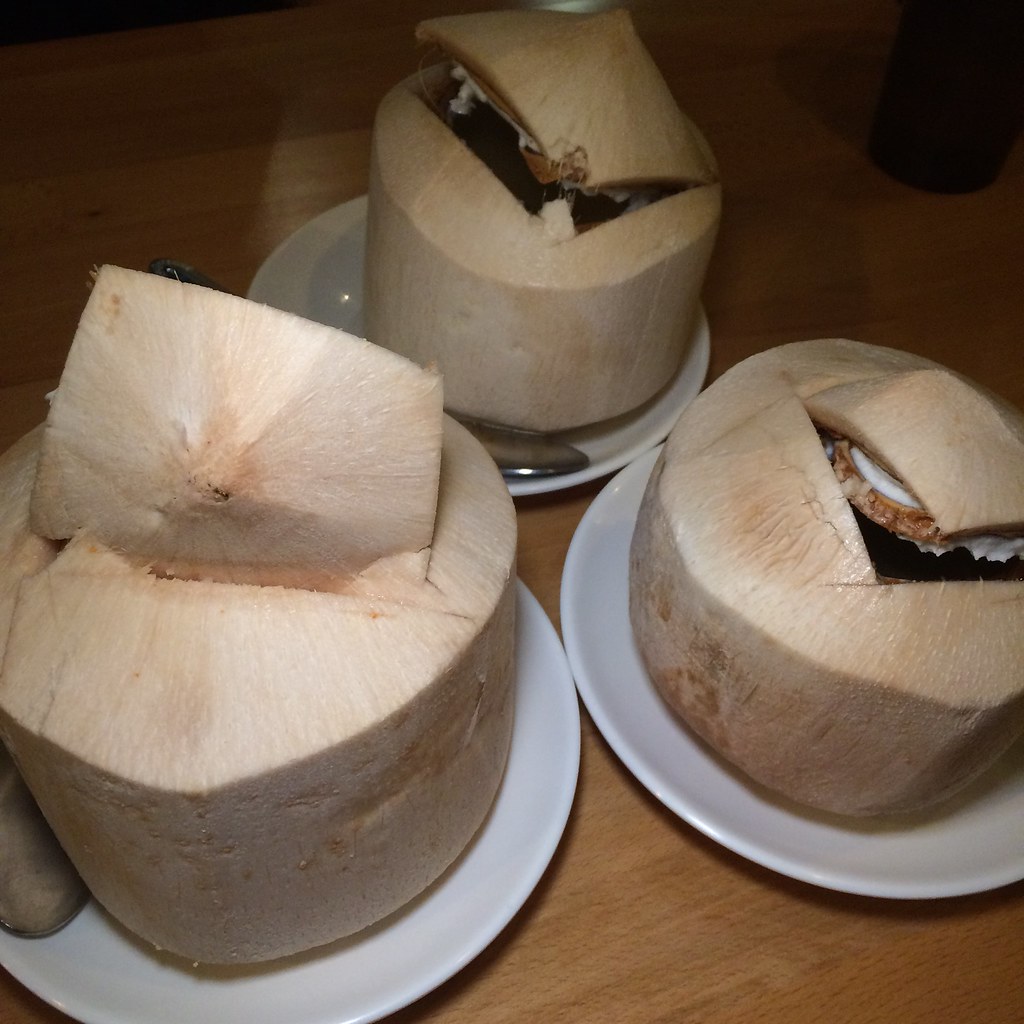This is a close-up photograph of three coconuts meticulously arranged on white ceramic plates, resting on a light brown wooden table. The coconuts, mostly tan with patches of light brown where remnants of the skin remain, have had their tops cut off to reveal their interiors. Each coconut has a large, square-like cutout showcasing a dessert-like filling, which combines the coconut's natural white and chocolate gray interior. The one on the right displays this white and chocolate gray interior prominently. Metal spoons are placed on the plates adjacent to the coconuts, with the one at the back clearly visible. The image, taken with a flash, illuminates the coconuts and plates, though the back portion of the image is less distinct, featuring a black cylindrical object. The overall presentation suggests that these coconuts have been cleaned thoroughly and possibly stuffed with a creamy dessert.